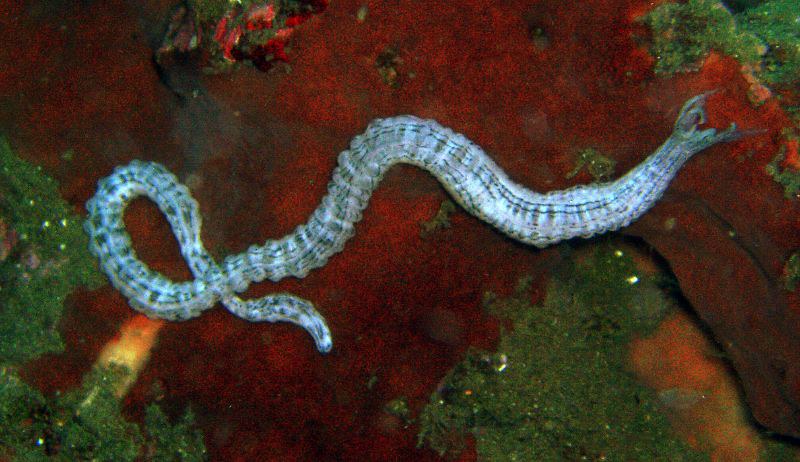The image depicts a scene predominantly set in shades of dark red, suggesting it might be the bottom of an aquarium or a shallow body of water. Central to the image is a slender, long creature resembling a sea snake. This creature is light blue with dark streaks along its back. Its body starts from the left side, curls elegantly, and stretches out diagonally to the upper right corner. Surrounding the sea snake, there are hints of green, possibly algae or aquatic plants, visible on the left side, at the bottom, and in the upper right corner, adding contrast to the red background. The backdrop contains various hues including green, orange, and a touch of yellow, suggesting rocks or corals. The overall composition appears as if captured through a close-up or microscope, highlighting the detailed, translucent texture of the snake-like organism. The creature’s mouth, positioned towards the upper right, seems to split open prominently, resembling a characteristic of predatory worms, evocative of the sandworms from Dune or the creatures from Tremors.